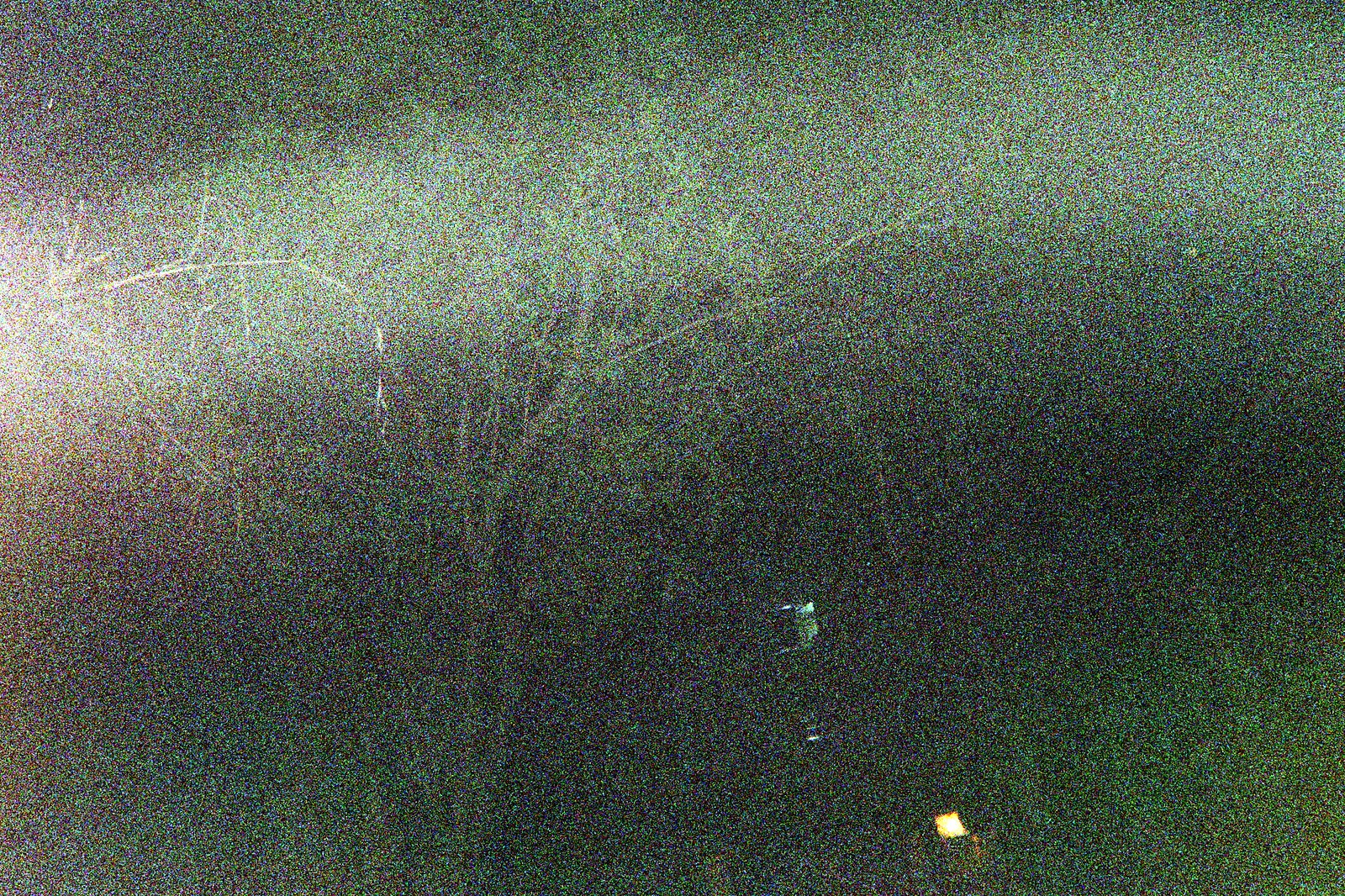This image appears to be an extremely grainy and abstract night photograph taken outdoors. The main feature is a dark green tree extending vertically from the left side of the image, with multiple trunks and horizontal branches forming a sparse canopy. The tree, along with the entire photo, is rendered in low resolution, adding to the grainy texture with small black and gray granules spread throughout. To the left of the tree, a bright flash of light with white and orange accents emanates, resembling the effect of an old Polaroid picture. There is also a distinct yellow, squarish light in the lower part of the image, which could be coming from a man-made source like a car, lantern, or street post. The background features a dark sky with some hints of green, possibly indicating a tree line. Overall, the image’s graininess and scattered lights give it an abstract, almost art-like quality.